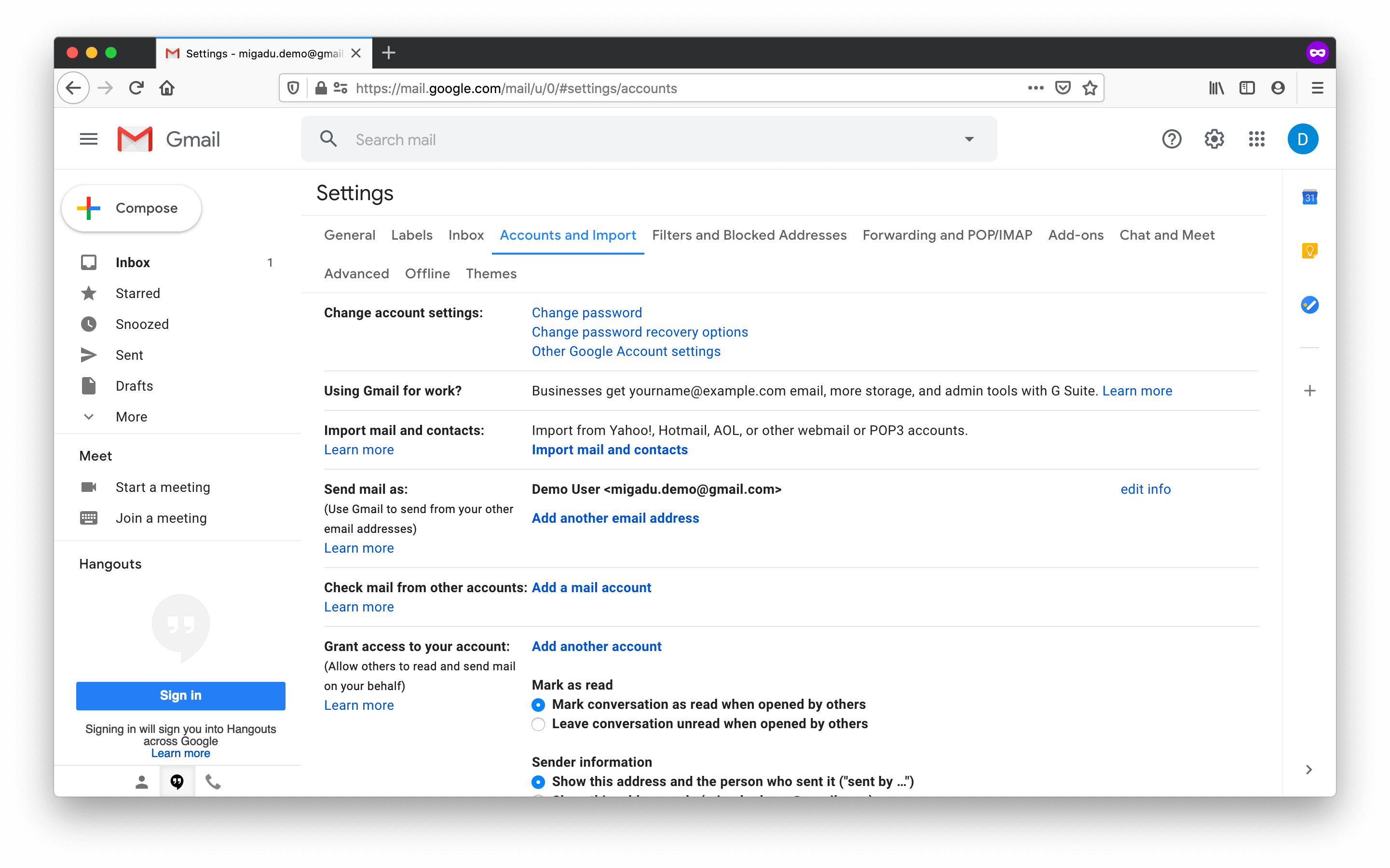This desktop screenshot, taken from a MacBook or an Apple desktop product (indicated by the iconic red, yellow, and green dots in the upper left corner), showcases the Gmail settings page, specifically focusing on the "Accounts and Import" settings. The webpage is displayed in light mode, and although the user is seemingly signed into their Google account (evident from the top-right corner), they are not signed into Gmail itself. 

The Gmail interface includes the standard hamburger menu button next to the logo, alongside buttons for composing an email, and navigating through folders such as Inbox, Starred, Snoozed, Sent, Drafts, and More. Below these options, there are buttons for starting or joining a meeting, indicating integration with Google Meet. The Hangouts menu appears empty in this screenshot.

The settings section is concise and orderly, listing tabs for General, Labels, Inbox, Accounts and Import, Filters and Blocked Addresses, Forwarding and POP/IMAP, Add-ons, Chat, and Meet. However, due to the screenshot being compressed and the text rendered somewhat unreadable, the specific details of the settings remain unclear.